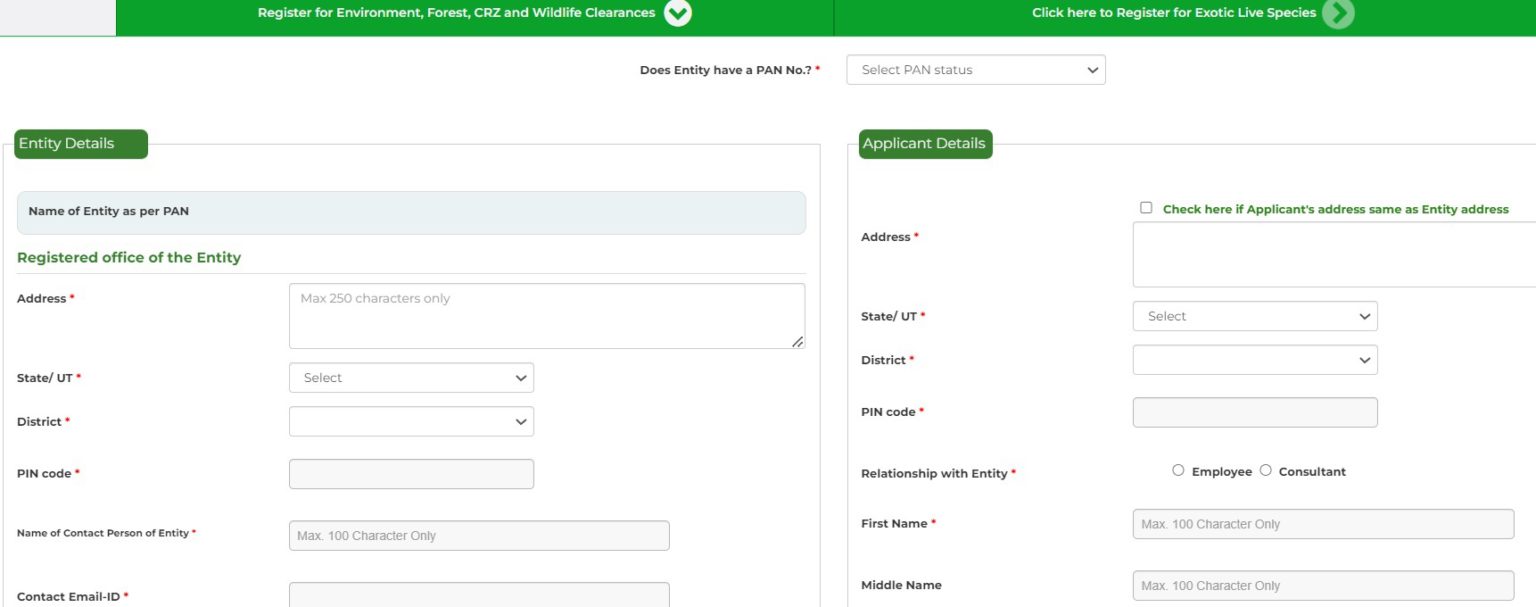This image appears to be a screenshot from a conservation website focused on registration for environment, forest, CRC, and wildlife clearances. The top of the image features a prominent green header with the text "Register for Environment, Forest, CRC, and Wildlife Clearances," along with a clickable prompt to register for exotic live species. 

On the left side of the image, there is a green form labeled "Entity Details." This form includes fields for entering the "Name of Entity as per PAN," "Registered Office of the Entity," "Address," "State," "District," "Pin Code," "Name of Contact Person or Entity," and "Contact Email."

On the right side, another section titled "Applicant Details" is present. This section includes fields for entering the "Address," "State," "District," "Pin Code," and "Relationship with Entity." There are also spaces for "First Name" and "Middle Name" of the applicant. Below these fields, there are checkboxes that allow the applicant to indicate if their address is the same as the entity's address and to specify if they are an "Employee" or "Consultant." 

Additionally, above these sections, there is a form question asking "Does Entity Have a PAN Number?" (P-A-N). Overall, the website's main color scheme is white and green, aligning with its conservation-focused theme. 

This detailed image captures the structured and organized layout of the registration process, emphasizing the importance of accurate and thorough information for conservation efforts.